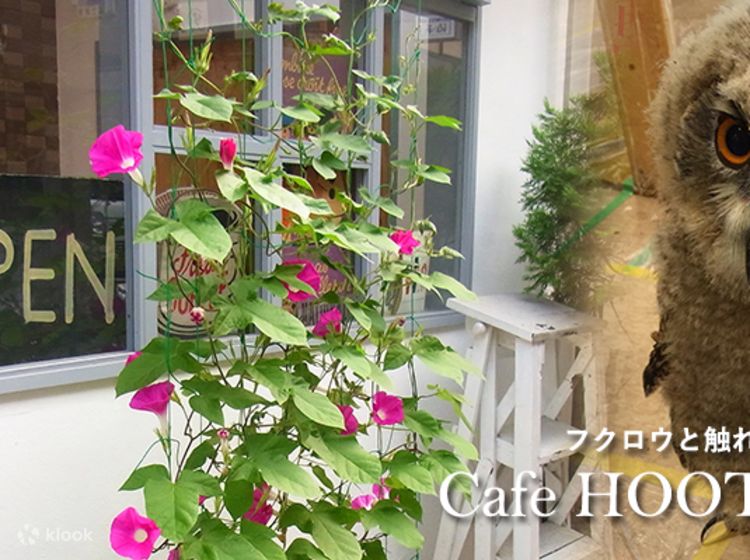The image depicts the exterior of a cafe called "Cafe Hoot." Dominating the left side of the image is a trellis adorned with green vines and oval-shaped leaves, punctuated by distinctive flowers. These flowers have white tubular bases that expand into pink petals, exhibiting a purplish-pink hue. Behind the trellis, a large glass window with a gray frame displays a black sign with handwritten text partially visible as "EN," likely indicating "open." A white stepladder is positioned next to this window. To the right, the image captures a close-up of an owl, revealing only half of its eye and part of its facial feathers, suggestive of a thematic connection to the cafe. The overall image appears to be a cropped flyer for the cafe, with additional textual details at the bottom mentioning "Cafe Hoot," alongside partially visible text in an Asian language. The interior glimpses hint at brick walls, contributing to a cozy atmosphere of the cafe.